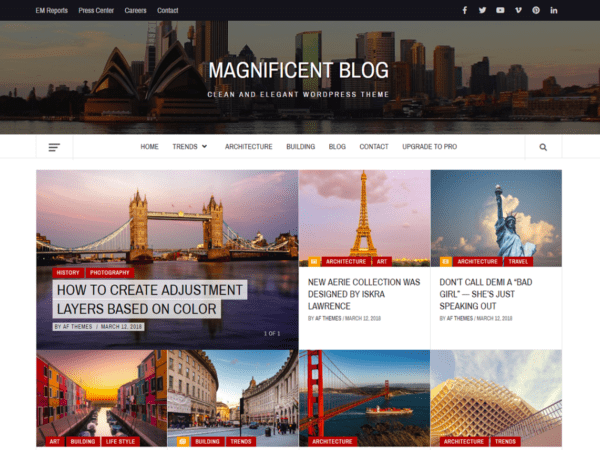This landing page showcases the "Magnificent Blog," a clean and elegant WordPress theme. At the top, an enticing header image features a city skyline against a sky backdrop, overlaid with the blog’s title "Magnificent Blog" and the tagline "Clean and Elegant WordPress Theme." Just beneath this, a navigation bar presents seven categories: Home, Trends, Architecture, Building, Blog, Contact, and an option to "Upgrade to Pro."

Below the navigation bar, the layout features several articles, each represented by captivating images. The first image, depicting a bridge in Britain, leads to an article titled "How to Create Adjustment Layers Based on Color," tagged under History and Photography. The second prominent image highlights the Eiffel Tower, leading to an article entitled "New Aerie Collection Designed by Iskra Lawrence." The third image showcases the iconic Statue of Liberty with a cloudy sky, linked to an article titled "Don't Call Demi a Bad Girl, She's Just Speaking Out."

Additionally, there are four more images serving as placeholders without headlines. One features the vibrant Piccadilly Circus in London, while another shows the majestic Golden Gate Bridge in San Francisco. The two remaining images, though not immediately identifiable, presumably depict other famous international landmarks.

These sample articles and images illustrate the theme's aesthetic and functionality, demonstrating how vibrant and visually appealing a blog can be when utilizing "Magnificent Blog" on WordPress.